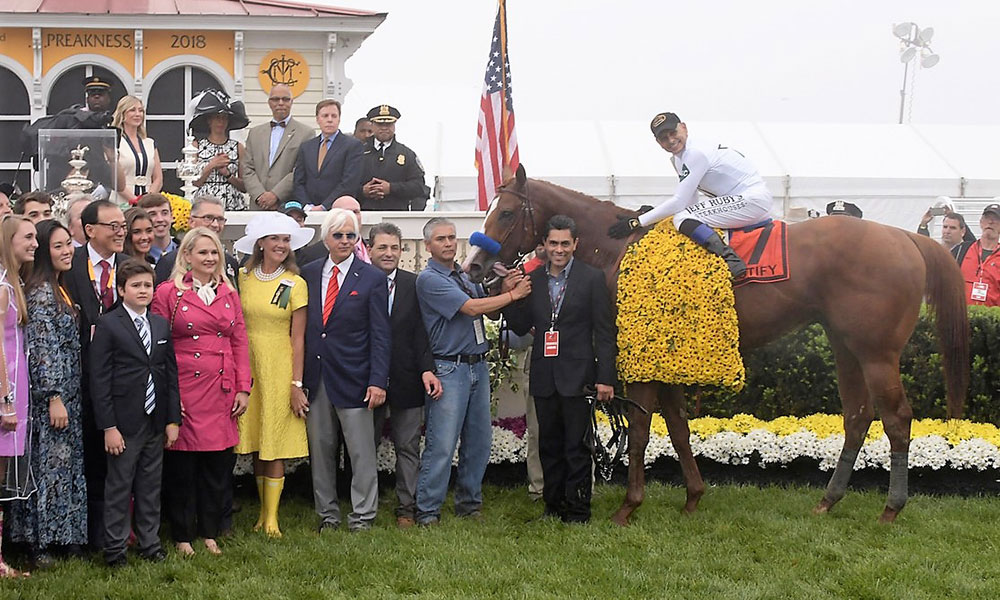In this horizontally rectangular, full-color photograph taken outdoors on an overcast day, a jubilant scene unfolds in front of a community center. The image, devoid of borders or backgrounds, captures a triumphant moment at a horse racetrack. Central to the scene is a majestic brown horse adorned with a drape of yellow flowers, indicating a significant victory. The jockey, dressed in a white uniform and black helmet, sits proudly atop the horse, which bears the number "7" on its blanket.

Surrounding the horse and rider is a celebratory crowd dressed in various attires - men in suits, jeans, and pants of grey and black hues, and women in brightly colored gowns. The diverse gathering exudes joy, likely stemming from the recent win at the event prominently marked as "Preakness 2018," evident from the text on the building and a fluttering American flag above the horse's head.

In the background, a glass case holds a gleaming gold trophy, further attesting to the horse's victory. Amidst the crowd, at least one security person is visible, ensuring the occasion's orderliness. The color palette of the photograph features a vibrant mix of blue, black, green, yellow, pink, white, red, and various shades of green, combining to visually represent the festivity and grandeur of the event.